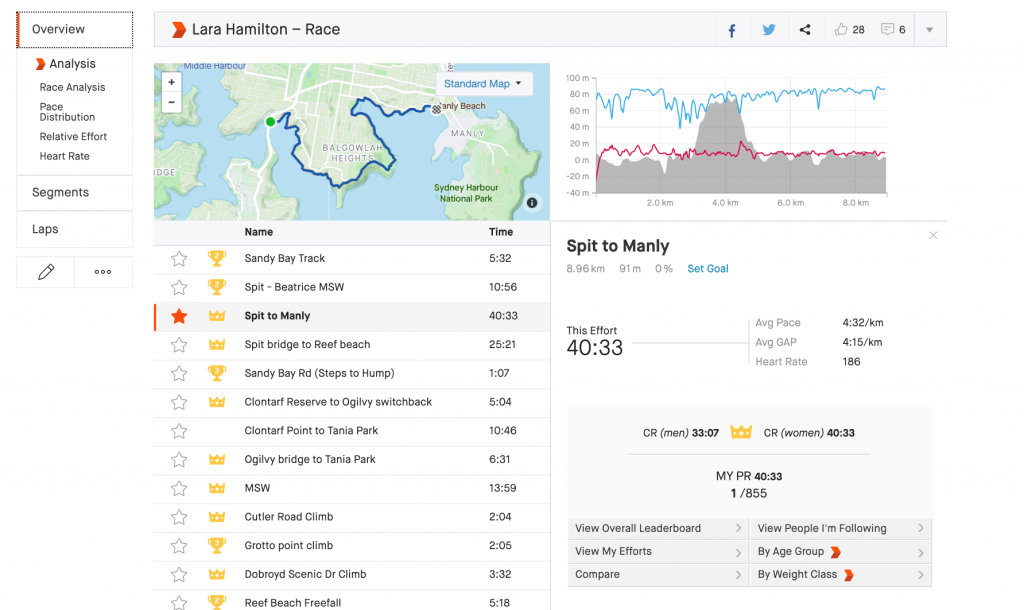**Detailed Caption:**

This screenshot from the fitness tracking application Strava showcases an in-depth analysis of Lori Hamilton's recent run or race. The user interface is sectioned into several parts: on the left navigation menu, options like "Overview," "Analysis," "Race Analysis," "Pace Distribution," "Relative Effort," "Heart Rate," "Segments," and "Laps" ensure comprehensive data accessibility. The central part of the screen prominently features a map displaying the route taken, traced in a blue line, beginning at Sandy Bay Track and navigating through key landmarks such as Balgo Wall Heights and Sydney Harbor National Park, before finishing at Manly. 

Key segment times are detailed:
- Sandy Bay Track: 5:32
- Spit to Beatrice MSW: 10:56
- Spit to Manly: 40:33

The final segment time, highlighted with a star, signifies its importance with this specific race. Other notable segments include Spit Bridge to Reef Beach, Sandy Bay Road, and Klon Tarf Reserve, noted alongside their respective timings.

Furthermore, the screenshot contains a performance graph, detailing pace and heart rate fluctuations throughout the race. Social sharing features are also accessible, with icons for platforms like Twitter, allowing for personal achievements to be shared easily. Overall, the image provides a detailed evaluation of Lori Hamilton's race performance, from route specifics to segment analyses, personal record highlights, and available social sharing options.